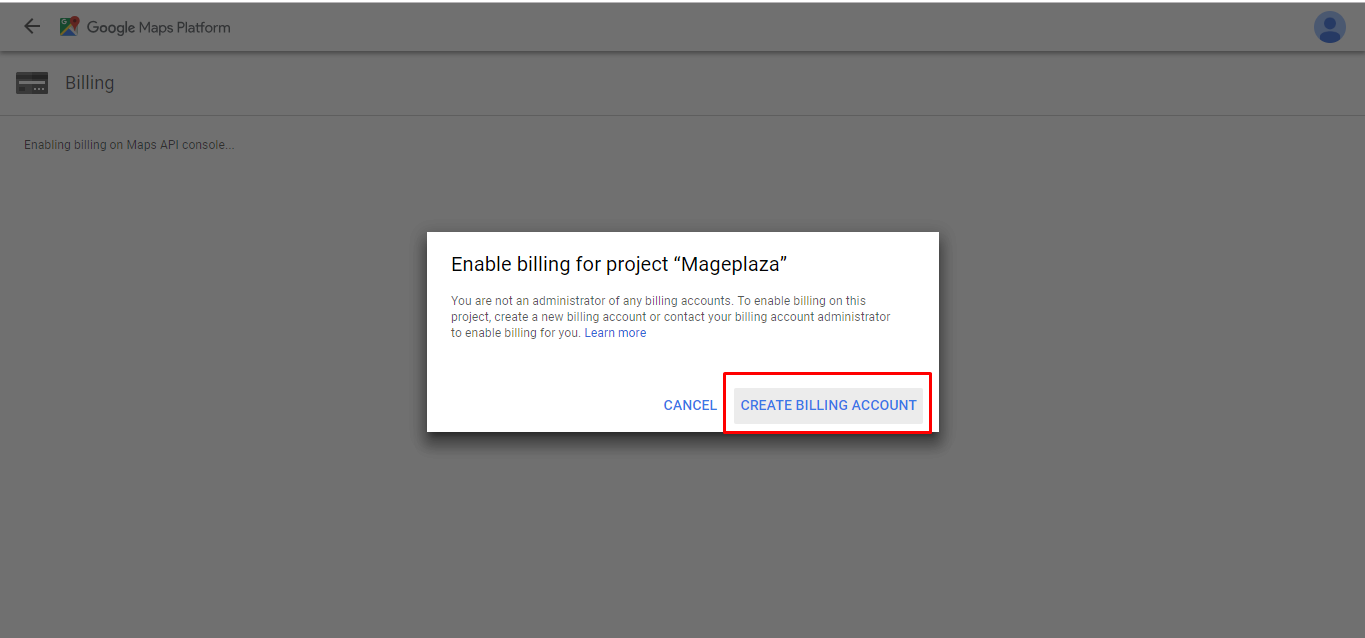The screenshot depicts a section of the Google Maps Platform user interface. 

In the top-left corner, there is a "Google Maps Platform" label accompanied by a left-arrow icon. On the far-right side of the upper section, there is a generic profile circle icon. Below this header, a gray horizontal line divides the screen. 

Directly underneath the gray line is a "Billing" tab. Below this tab, the text within the screen is small and difficult to read. The main content below this is a pop-up menu containing the following message: 

"Enable billing for project 'Made Plaza.' You are not an administrator of any billing accounts. To enable billing on this project, create a new billing account or contact your billing account administrator to enable billing for you."

The pop-up menu includes links labeled "Learn More" and a blue "To Enable" button. Beneath this are two additional buttons: a "Cancel" button and a "Create Billing Account" button, with the latter highlighted by a red rectangular box.